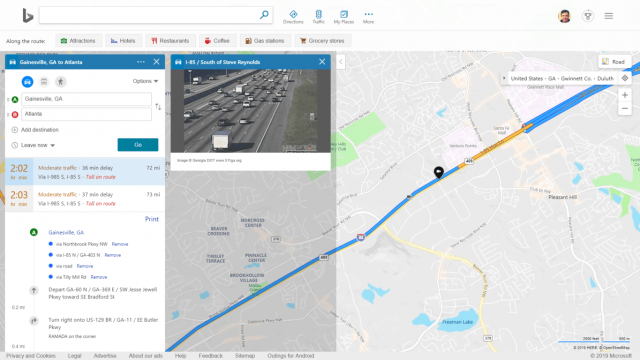"A screenshot from Bing Maps displays a detailed route from Gainesville, GA to Atlanta. The interface is organized into three distinct panels. The left panel features the starting point, Gainesville, GA, and the destination, Atlanta, along with a 'Go' button to initiate navigation. It also displays current traffic conditions and highlights various stops along the route. The middle panel showcases a live, black-and-white traffic camera feed of the highway, providing real-time traffic updates. The right panel presents the actual map with the route prominently highlighted in blue. A black location pin marks a midpoint on the journey. The Bing logo is visible at the top of the interface, indicating the map program is by Microsoft, not Google Maps."